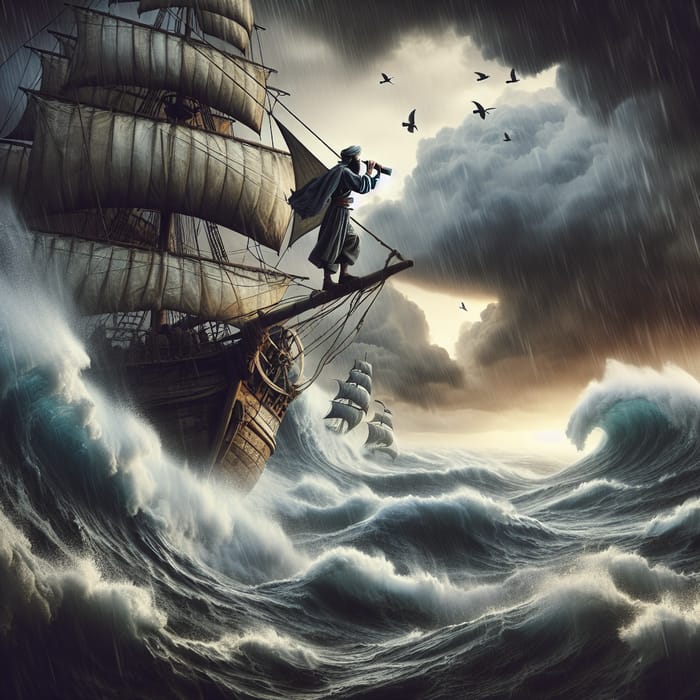The digital illustration depicts a stormy maritime scene with vintage ships, reminiscent of Spanish galleons or pirate vessels, navigating tumultuous, dark waves capped with white foam. In the foreground, a grand wooden ship, bearing numerous unfurled sails, battles against the rough seas. Atop a large rectangular mast extending from the ship’s front, a man garbed in a flowing blue cape, puffy pants, and a blue turban reminiscent of Aladdin, stands braving the fierce wind. He peers through a telescope, scanning the horizon. His cape billows dramatically in the storm. The sky is ominously dark, filled with thick, black clouds, and the pallid, golden-hued light near the horizon is pierced by seven silhouetted birds. In the distance, two more ships, similarly rigged with large sails, struggle through the relentless storm, which is punctuated by lines of rain and a curling tidal wave on the right. The artist's attention to detail brings the chaotic energy of the storm to life, capturing the peril and determination of the scene.